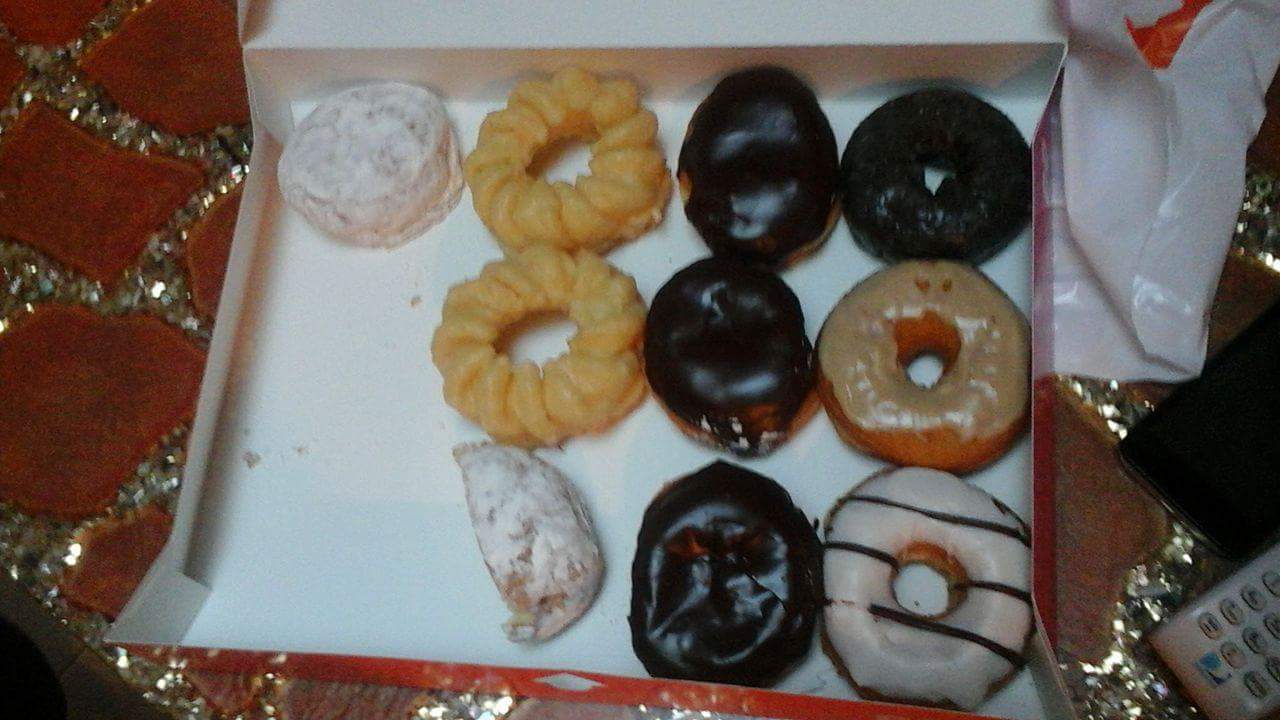This photograph captures a top-down view of an open, flimsy reddish cardboard box designed to hold twelve doughnuts, arranged in four rows of three. Currently, it contains nine and a half doughnuts, with the missing pieces suggesting some have been eaten. Each doughnut is distinct: in the upper right corner, there's a black doughnut followed by a brown maple-flavored one with light beige icing. Below that, a doughnut with white icing and three vertical brown bands stands out. The next row features three identical thick, cream-filled doughnuts with brown icing. Moving downward, there's a light brown cruller followed by another similar cruller and half of a white powdered doughnut. The bottom row contains a single, full white powdered doughnut, leaving space for two more that are no longer there. The box sits on a red table with a gold square design, and a remote is visible at the lower right corner of the image.